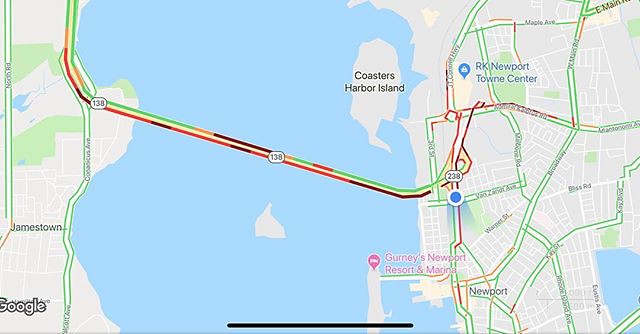This image features a detailed Google map, prominently displaying a large blue waterway that separates two main land masses with distinct labels and locations. To the left, you briefly see the outline of Jamestown. Spanning across this waterway is a bridge labeled 138 on the left side and 238 on the right, further connecting the islands. On the right, the expanse is more detailed, highlighting several critical areas such as Newport with notable locations like RK Newport Town Center and Gurney's Newport Resort and Marina. Additionally, a smaller land area identified as Coasters Harbour Island appears at the upper part of the image, adding to the map's complex geographical information. The map also includes various roadways, marked with white and green lines, showcasing the intricate network of streets that bind these places together. At the bottom of the map, the familiar Google logo is visible, confirming the map's source.